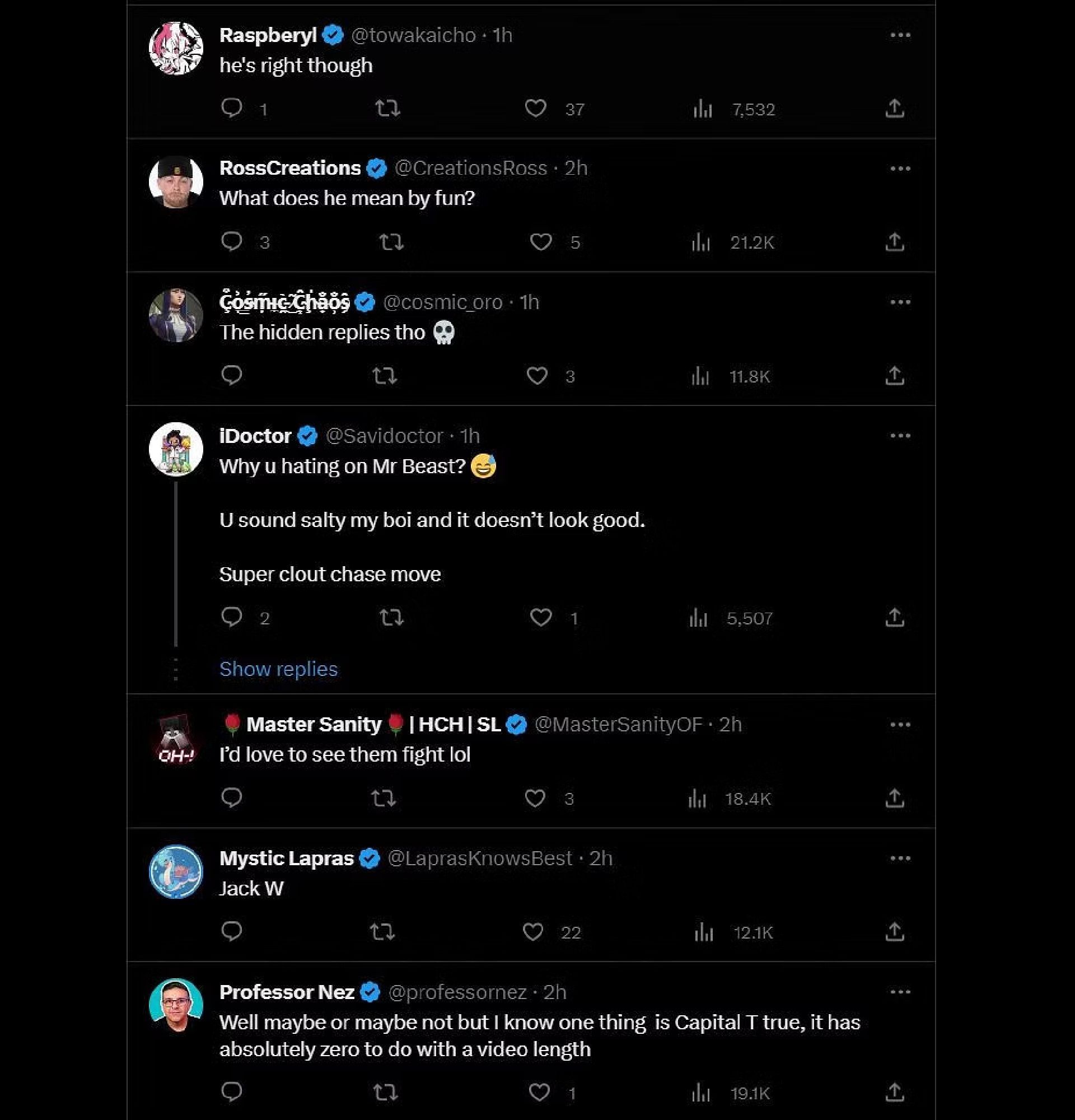This image features a large black square as its background. At the top, it showcases the username **"Razz Beryl"**, accompanied by a verified Twitter logo with a check mark and an icon representing Razz Beryl. To the right of the username, there are three horizontal dots symbolizing additional options.

Below this, an interaction between different Twitter users is depicted:

1. **Razz Beryl**: "He's right though." (written in white text)
2. **Ross Creations**: Username "Creations Ross - 2H" with a profile picture of a man wearing a cap. To the right, there are three horizontal dots. The tweet reads: "What does he mean by fun?"

Next, there is a tweet from **Gothic Chaos** with the handle "@cosmic_ORO-1H", illustrated with a circular profile picture of a girl. To the right, there are three horizontal dots. The tweet reads: "The hidden replies though 💀".

Following, there is a user named **iDoctor** with a user icon and no additional text provided.

Subsequently, **Master Sanity** comments: "I'd love to see them fight lol."

Then, a user named **Mystic Lapras** appears without additional information.

Finally, **Professor Nez** with the handle "@ProfessorMez" provides a detailed statement: "Well, maybe or maybe not, but I know one thing is TRUE, it has absolutely zero to do with video length."